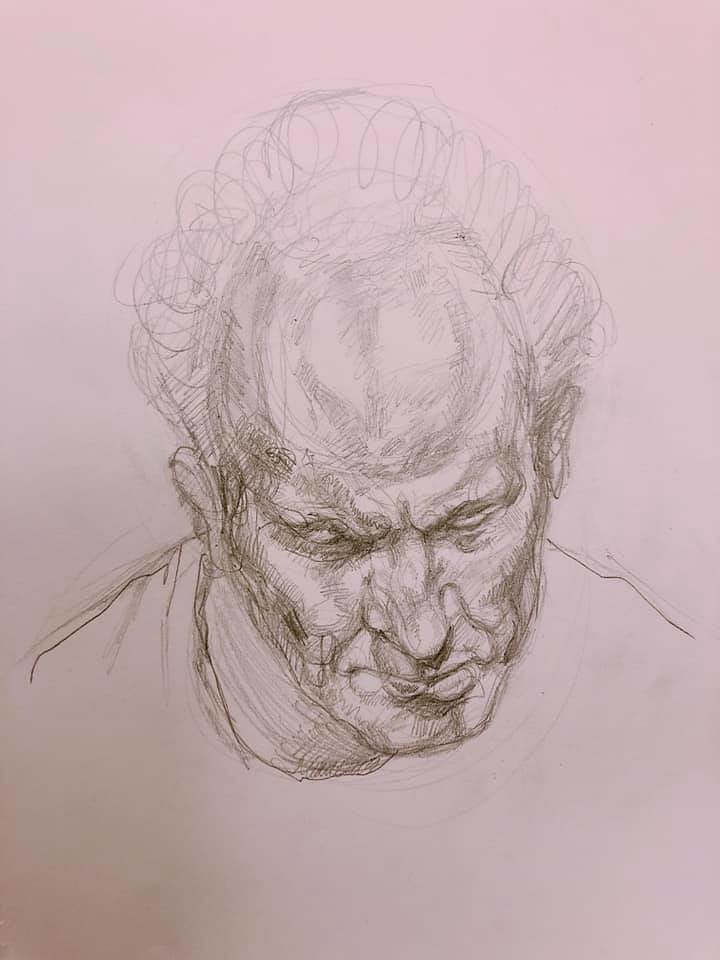This meticulously detailed pencil sketch portrays a contemplative elderly man, characterized by his balding head with tufts of curly hair encircling the sides and back. His downcast gaze conveys a pensive mood, further emphasized by his deeply furrowed brow. The artist has employed adept shading techniques, particularly across the man's face, to accentuate the hollows beneath his pronounced cheekbones. His prominent nose, thin upper lip, and square chin contribute to the distinctiveness of his features. The man is dressed in a simple crew neck shirt, with subtle evidence of erased pencil marks around its neckline, suggesting a thoughtful and deliberate creation process.